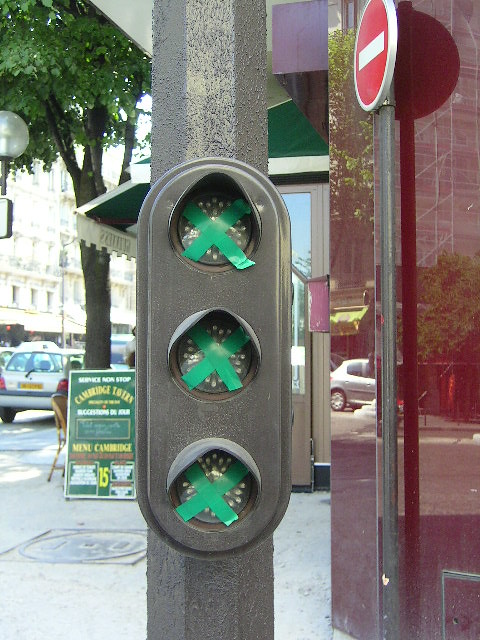The photograph, taken outdoors on a sunny day, prominently features a non-functioning traffic light mounted on a metal pole in the center. The traffic light has three circular lights aligned vertically, each covered with green tape forming an 'X'. To the right, there's a shiny red wall reflecting automobiles and displaying a metal pole with a red circular prohibition sign featuring a horizontal white line. In the upper left corner, a multi-story white building with numerous windows is visible, partially obscured by tree foliage with bright green leaves. Below, a road lined with cars, including a noticeable white car, and a sidewalk can be seen. A sign is present in front of the tree, and a manhole cover, appearing slightly left of center at the bottom, adds further detail to the street scene.